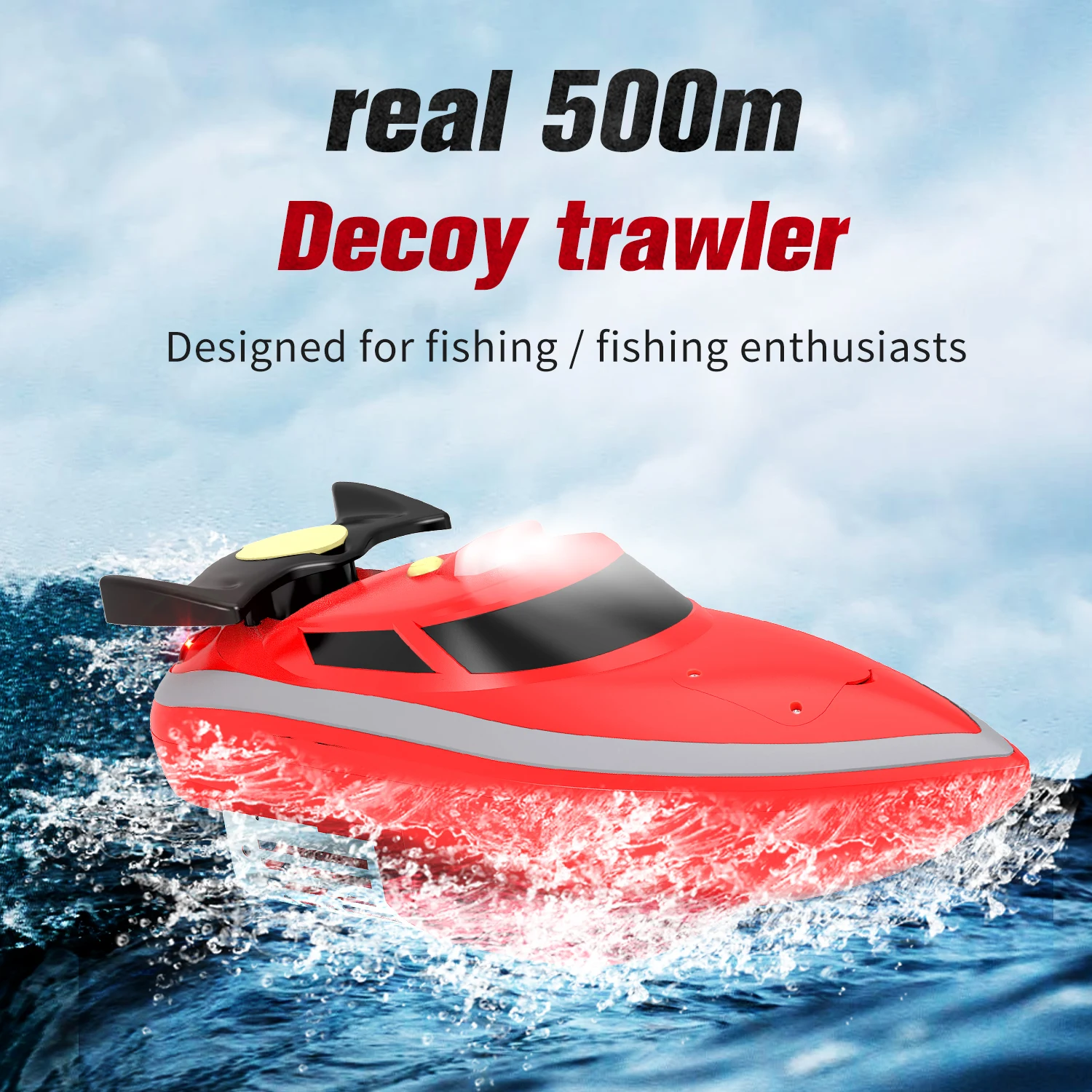The image appears to be an advertisement or poster with a squarish shape, depicting a boat that looks like a toy boat. The boat featured is a small, red speedboat with a gray stripe running along its side. It has a distinct roof with dark windows and a black motor or spoiler at the back. The boat seems to be traversing a body of water, creating splashes below its hull. The background showcases a light blue sky accented with white clouds. Prominently displayed at the top of the illustration is the text "Real 500m" in bold black font, and directly beneath it, "Decoy Trawler" in red font. Further down, in smaller black text, it states "Designed for fishing/fishing enthusiasts." This gives the impression that the boat, despite looking like a toy, might be a real boat designed for fishing aficionados.